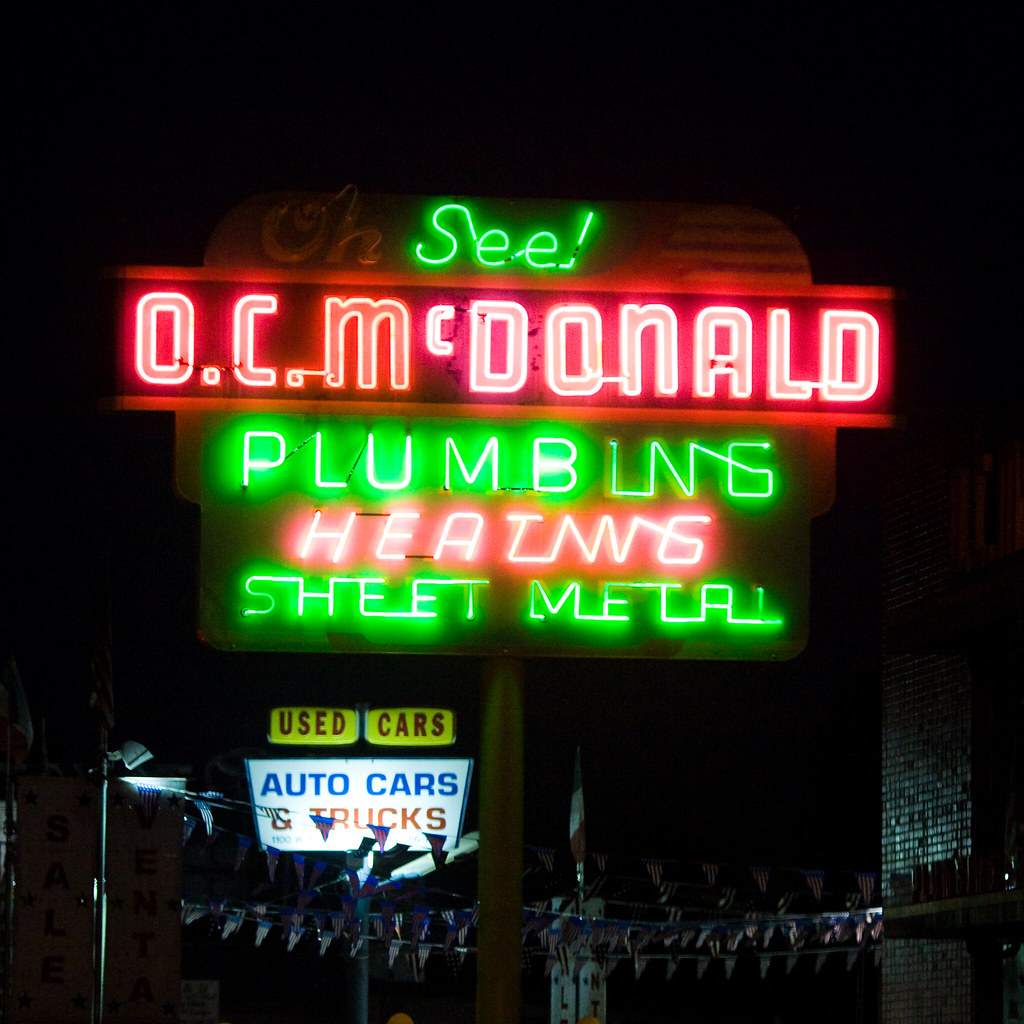In the photograph, a neon sign is prominently displayed against a backdrop of darkness, making it the focal point of the image. The sign reads "OC, McDonald, Plumbing, Heating, Sheet Metal" in vibrant neon colors. However, the letter "O" is not lit, creating a noticeable contrast. The words "C," "Plumbing," and "Sheet Metal" glow in green neon, while "OC," "McDonald," and "Heating" are illuminated in pink neon. The sign has a unique shape, rounded at the top and more squared off through the rest of it. Below this main sign, there is another sign that reads "Used Cars, Auto Cars, Trucks," adorned with red, white, and blue American flags. On the bottom left, a street sign can be seen along with another sign that says "SAILVENTA." To the right, there's a brick or stone building, barely visible in the nighttime darkness. Although it is night, the neon lights add a vibrant burst of color to the scene, subtly illuminating the surrounding area.